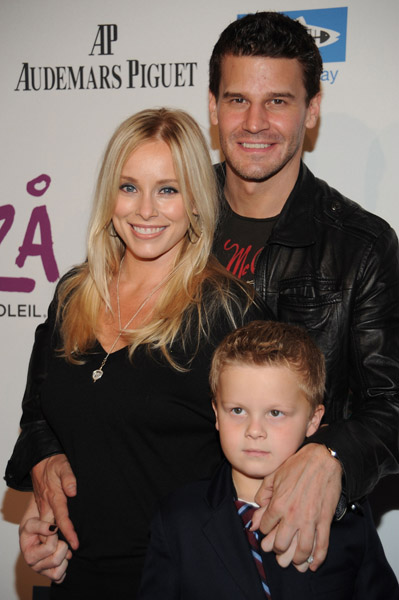The image depicts a well-known actor, likely David Baran from the show "Bones," posing for a family photo with his wife and son against a white backdrop displaying "AP Audemars Piguet." The actor, who has brown or dark hair, is dressed in a black jacket over a black shirt featuring a red letter 'M' and other text. He is smiling warmly at the camera. His wife, standing to his right (our left), is shorter, sporting long blonde hair parted in the middle, and adorned in a black top with a silver necklace that boasts a locket pendant. She too is smiling. Their son, appearing to be around seven to ten years old, has dirty blonde hair and a more serious expression, looking slightly away from the camera. The family seems to be participating in a photo shoot or a formal event, possibly a red carpet gathering. The actor has his left arm around his wife and his right hand resting on his son's shoulder, creating a close, affectionate pose.